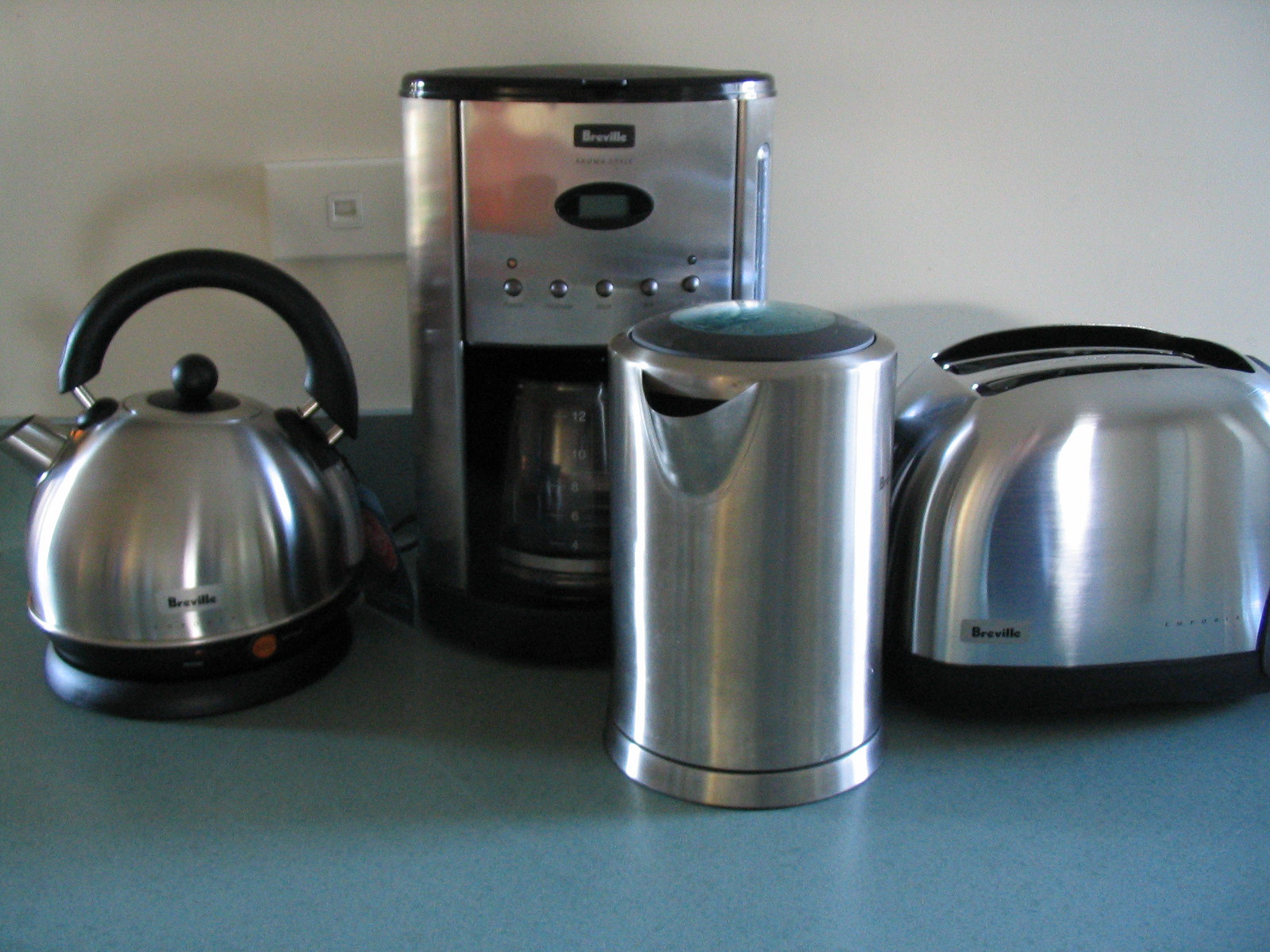The image showcases a collection of sleek, stainless steel kitchen appliances arranged on a bluish-green countertop set against a white wall backdrop. On the far left, there is a Breville electric tea kettle with a distinctive black plastic handle, round and contemporary in design, resting on a black base. To its right, there is a silver canister with a dark gray top, fitted with a spout presumably for dispensing tea or other liquids. Next to the canister, a contemporary Breville two-slice toaster is positioned, featuring a rounded design with a black base and two slots for bread. On the far right, a Breville coffee maker with a glass carafe is visible, equipped with multiple buttons and a digital display, showcasing a mix of stainless steel and black elements. This harmonious arrangement of modern appliances creates a clean, cohesive look in the kitchen space.